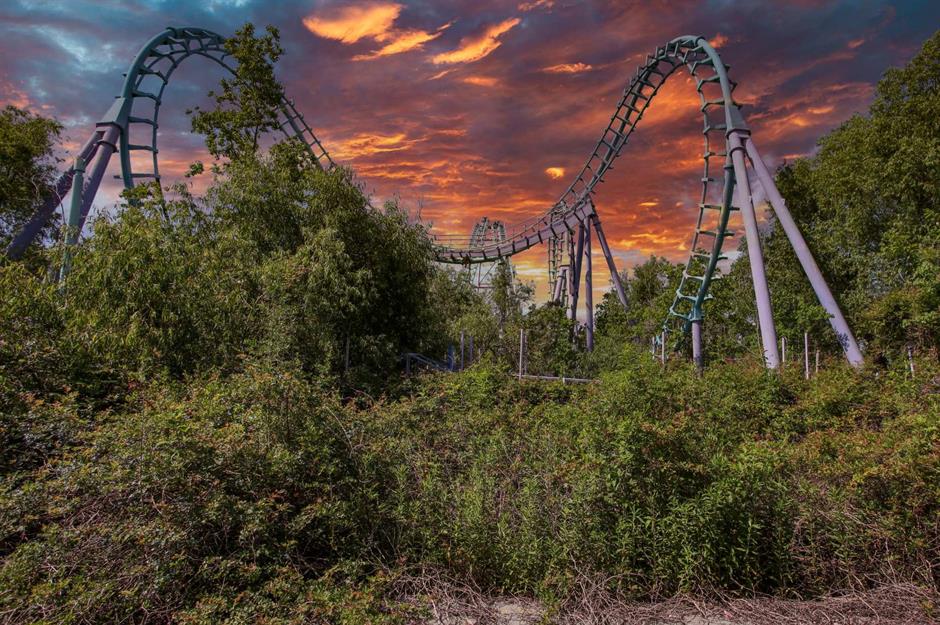In this image, possibly a photoshopped composite or an illustration, a deserted and deteriorating roller coaster is prominently featured. The metal structure, looping and seemingly falling apart, is overwhelmed by overgrown shrubbery that clings to and surrounds the ride. Two leaning metal stanchions suggest a once-functional but now crumbling apparatus. The foreground is dominated by chaotic plants and tall trees that almost entirely engulf the scene. In the background, an eerie and stormy sky intensifies the apocalyptic atmosphere, characterized by hues of reds, yellows, and blues, merging into purples and pinks, reminiscent of a dramatic sunset or a post-apocalyptic world. The stark contrast in lighting between the overgrown, desolate roller coaster and the vibrant, tumultuous sky lends an otherworldly feel to the image, as if depicting a world left behind by humanity.